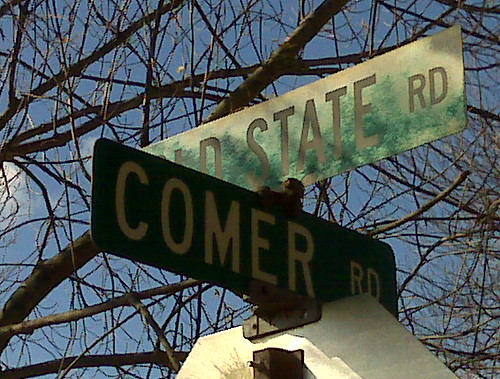The photograph captures two intersecting road signs positioned perpendicularly against a backdrop of a clear blue sky. Bare tree limbs, likely indicating a winter season, stretch across the sky. The image appears to be taken from a low angle, looking up at the signs. The lower sign, attached to the rear of a stop sign, is green and reads "Comer Rd," though it appears weathered with the green color faded significantly. The upper sign, running left to right, is partially obscured and also shows signs of significant wear, with the text likely reading "Old State Rd" or something similar, ending with "D State Rd." The overall appearance of both signs is faded, hinting at prolonged exposure to the elements.